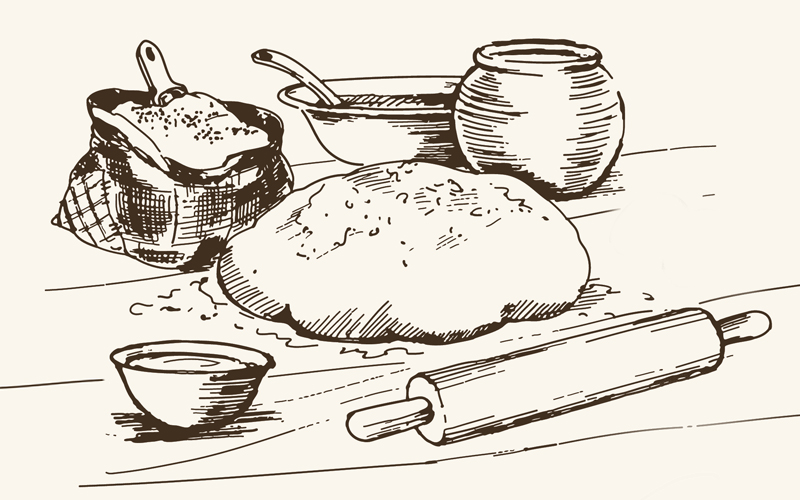This detailed black and white line art illustration, set against a cream background, depicts a collection of bakery items and utensils arranged as if on a cutting board. At the center of the image is a mound of dough, irregularly shaped and sprinkled with flour, ready for baking with spices dotted on top. Near the top of the illustration, a rounded bowl with a ladle is positioned to the left, accompanied by a rounded container, possibly pottery or glass, suitable for storing seeds or tea to the right of the bowl. On the top left, a sack of flour with a scoop inserted suggests the essential ingredient for baking. The bottom left features a small saucer filled with a liquid, possibly milk or eggs, while a rolling pin lies angled from the top right to the bottom left on the bottom right of the illustration, completing the scene. The entire composition evokes a sense of anticipation and preparation for baking, presented in a clean, line-drawn style. There is no identifying information about who created the drawing or the purpose behind it.